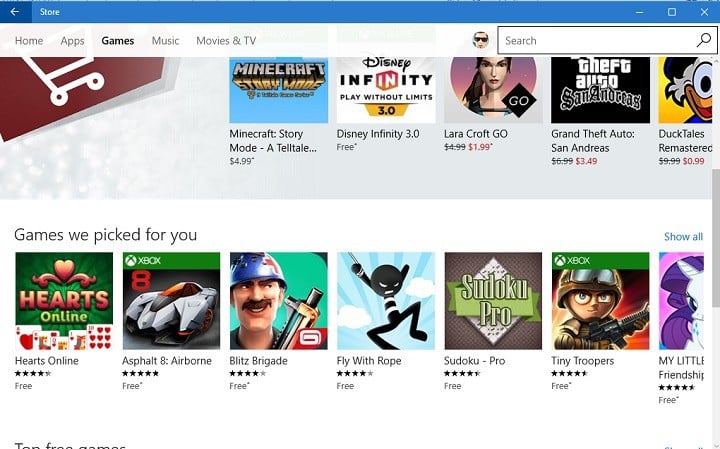This screenshot appears to be from an app store interface. The interface is dominated by a blue banner at the top featuring an arrow icon and the word "Store." Adjacent to the banner are icons for minimizing, maximizing, and closing the window (a dash, a square box, and an 'X', respectively). Below this are navigation categories including Home, Apps, Games, Music, Movies, and TV, with the Games category highlighted in a darker shade.

A search bar with a user icon for the search function is positioned prominently below the categories. The featured section under the search bar showcases a selection of games with vibrant icons. The games listed in this top row are: Minecraft Story Mode, Disney Infinity Play Without Limits 3.0, Lara Croft Go, Grand Theft Auto: San Andreas, and DuckTales Remastered.

The next section, titled "Games We Picked for You," is displayed on the left, with a "Show All" option on the right. This section presents another set of game icons, including: Hearts Online, Asphalt 8: Airborne, Blitz Brigade, Fly With Rope, Sudoku Pro, Tiny Troopers, and a partially visible title, likely My Little Friendship.

The image cuts off at the bottom, barely revealing a section titled "Top Three Games." The entire interface is set against a clean, white background, enhancing the visual appeal and legibility of the app store content.